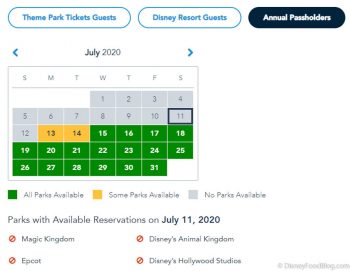The screenshot captured displays a central section of a user interface, likely from a tablet given its unique, almost square dimensions. The layout features no indicators for battery life nor time, which directs focus strictly to the content shown. 

At the top, there are three prominent, oval buttons labeled: "Theme Park Tickets," "Guests Disney Resort Guests," and "Annual Pass Holders." Below them, a large calendar is prominent, navigable via left and right arrows, currently set to July 2020. The calendar highlights various dates with color-coded availability status:

- **Gray (1st-12th):** No parks available.
- **Orange (13th-14th):** Some parks available.
- **Green (15th-31st):** All parks available.

The current date highlighted is Saturday, July 11th, 2020, boxed distinctively. Complementing this, a section at the bottom lists "Parks with available reservations on July 11th, 2020," specifying four parks: Magic Kingdom, Epcot, Disney's Animal Kingdom, and Disney's Hollywood Studios. The entire interface is set against a white background, giving it a clean and organized look.